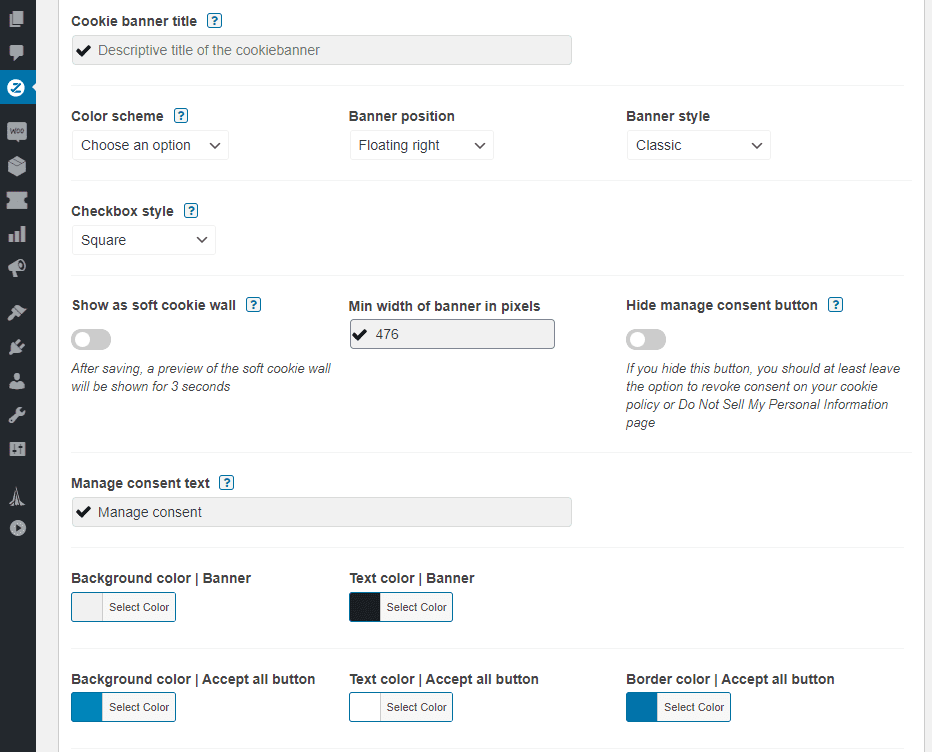This image displays a cropped screenshot of an online software panel for configuring a cookie banner. 

- At the top, it reads "Cookie Banner Title."
- Immediately below, there's a checkbox next to a text bar that states "Descriptive Title of the Cookie Banner."
- The section beneath this outlines various settings, starting with "Cookie Scheme" in bold black letters, followed by "Choose an Option" and a corresponding drop-down menu.
- To the right, "Banner Position" is set to "Floating Left," and "Banner Style" is designated as "Classic."
- Below this, there's a setting labeled "Show a Soft Cookie Wall" with an accompanying toggle switch currently set to off.
- Further down, there's a field for "Minimum Width of Banner in Pixels" which is set to 476.
- To the right, "Hide Manage Consent Button" also has a toggle switch that is in the off position.
- At the bottom, "Manage Consent Text" is filled in with "Manage Consent."
- Underneath, settings for appearance include: "Background Color Banner" set to gray, "Text Banner" set to black, "Background Color (Accept All Button)" set to blue, "Text Color (Accept All Button)" set to white, and "Border Color of (Accept All Button)" also set to blue.

This detailed configuration panel allows users to customize the visual and functional aspects of their cookie banner.